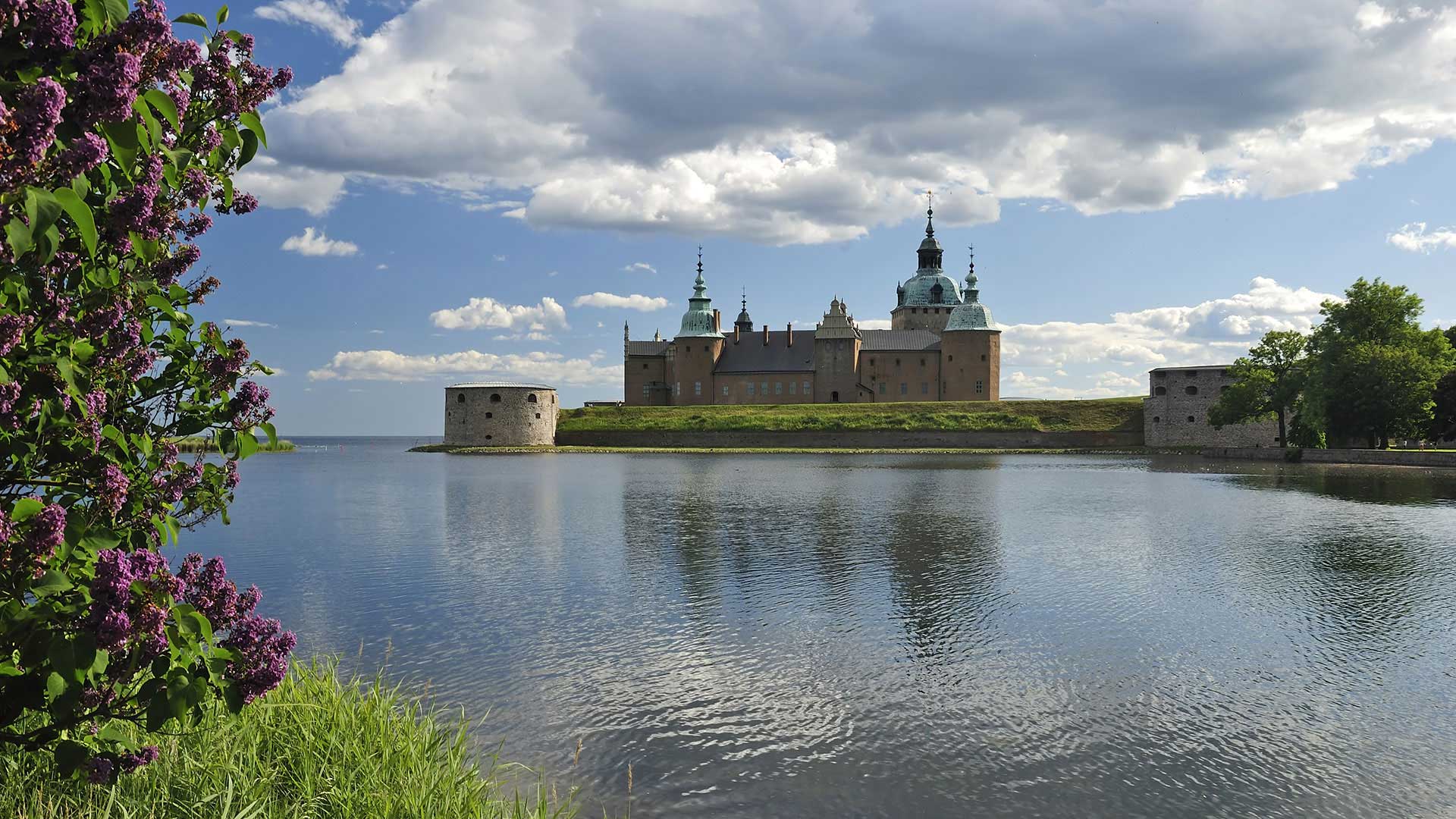This detailed photograph captures a picturesque scene of a large, ornate castle-like building situated on a verdant expanse of green grass, with a tranquil lake in the foreground. Dominating the center of the composition, the reddish-brick castle proudly rises with four metallic-looking spires and three chimneys on the front facade. Below and to the left of the castle, there is a smaller circular building with diminutive windows. To the right, a sturdy stone structure also features small circular windows, and is partly shaded by nearby trees.

The left side of the photograph showcases lush greenery adorned with vibrant purple flowers climbing from the bottom to the top. The sky above is a vivid blue, peppered with both large, dramatic clouds in the middle and smaller white clouds scattered around, casting a serene ambiance over the scene. The entire image is devoid of any visible people or animals, focusing entirely on the majesty and tranquility of the architectural and natural elements present.